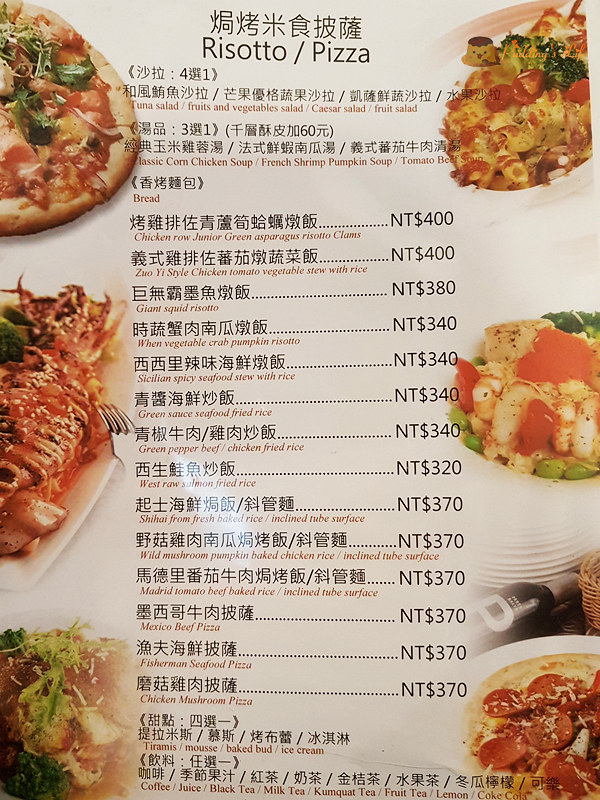**Menu Description for a Chinese Restaurant**

This menu, set against a whitish background, features a selection of dishes flanked by vivid food photos on both sides. At the very top, the menu is titled "Risotto / Pizza," with Chinese characters above each item translating both the names and descriptions of the dishes. 

The English translations for the dishes are listed beneath the Chinese text. In red, the menu offers a variety of salad options: Tuna Salad, Fruit and Vegetable Salad, Caesar Salad, and Fruit Salad. Following the salads are the soups: Classic Corn Chicken Soup, French Shrimp Pumpkin Soup, and Tomato Beef Soup, though part of this section overlaps with a food image, making it slightly difficult to read.

Below the soups, the menu lists:
- Bread
- Chicken Roe
- Junior Green Asparagus Risotto with Clams
- Zuo Style Chicken
- Tomato Vegetable Stew with Rice
- Giant Squid Risotto
- Vegetable, Crab, and Pumpkin Risotto
- Sicilian Spicy Seafood Stew with Rice
- Green Sauce Seafood Fried Rice
- Green Pepper Beef / Chicken Fried Rice
- West Raw Salmon Fried Rice
- Shiitake Fresh Baked Rice / Inclined Tube Surface (chef's special preparation)
- Wild Mushroom Pumpkin Baked Chicken Rice / Inclined Tube Surface
- Madrid Tomato Beef Baked Rice / Inclined Tube Surface
- Mexico Beef Pizza
- Fishermen’s Seafood Pizza
- Chicken Mushroom Pizza
- Desserts including Tiramisu, Mousse, Baked Bud, and Ice Cream
- Beverages such as Coffee, Juice, Black Tea, Milk Tea, Kumquat Tea, Fruit Tea, Lemonade, and Coca-Cola (explicitly written as Coca-Cola).

The left-hand side of the menu features a series of food images illustrating some of these dishes:
1. At the top left, a pizza garnished with greenery and a reddish topping.
2. Below that, a seafood dish with tantalizing tentacles on a white plate, accompanied by a fork.
3. Next, a possibly pinkish dish, perhaps fish or prosciutto, accented with fresh greenery.
  
On the right-hand side, the images include:
1. At the top right, a pasta dish adorned with broccoli and tomatoes on a white plate.
2. In the center, shrimp with hints of pink (possibly fish) and greenery such as edamame on a white plate.
3. At the bottom, a flatbread pizza topped with pepperoni and possibly sprinkled with Parmesan cheese, placed on a white plate. Between this plate and the one above, there’s part of a basket and a black bottle with a gray label featuring a bold white "P".

This detailed menu not only lists an extensive array of dishes but also provides a visual feast, giving potential customers a glimpse of the restaurant’s diverse offerings.